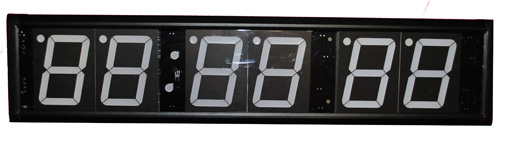The image showcases a sleek digital clock that is currently turned off, set against a plain white background. The clock itself is long and rectangular, framed by a black border that appears to be made of either plastic or metal, giving it a smooth, modern finish. The clock's face is also black, and though it is not illuminated, the structure of the digits is visible. Each number is displayed as '88', indicating that the segments are not currently active. The digits are arranged in three sets of two numbers each, separated by small, circular dots that likely serve as time separators. These dots are colored in a pale silver hue, adding a subtle contrast to the overall design. The digits themselves are a light, purplish-gray color, almost resembling lavender, and each number has a tiny dot positioned in the upper left-hand corner. This understated detail contributes to the clock's contemporary aesthetic.